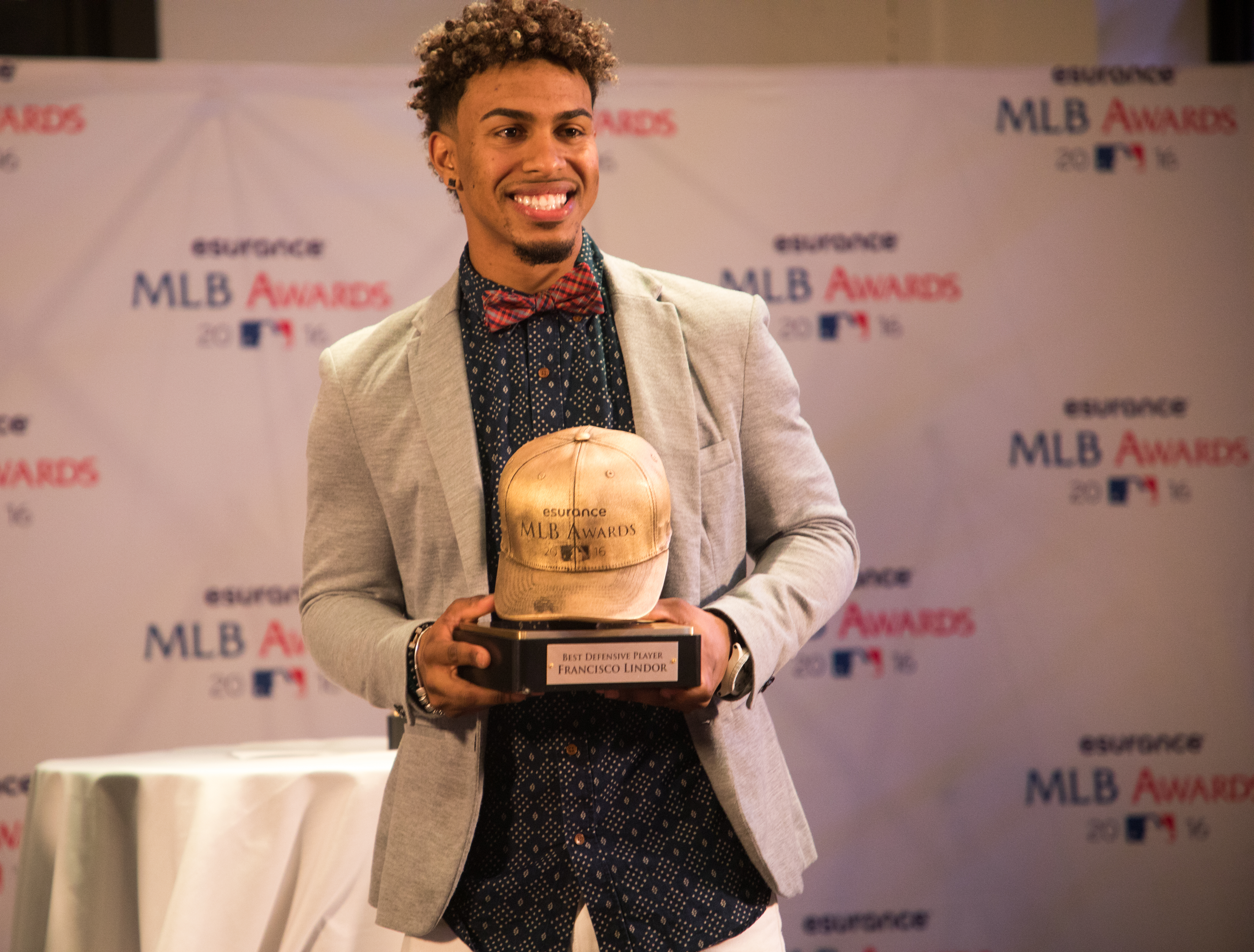In this vibrant image, the scene is set against an MLB Awards backdrop presented by eSurance, featuring a repeating Major League Baseball logo and partially obscured text. The foreground captures a young African-American man, positioned just slightly left of center, holding an award with a proud smile as he looks directly at the camera. He sports curly brown hair, a light beard, and a mustache, complemented by a light-colored suit jacket over a dark shirt adorned with white designs. A reddish bow tie adds a touch of flair, and though his shirt appears untucked at the bottom edge of the image, his confidence shines through. The award, held with both hands, features a brown base with an unreadable plaque, topped by a golden or brass baseball cap, also inscribed with illegible text. Adding to his distinguished look, he wears a watch on his left wrist and bracelets on his right. The image is sharply focused on the man, while the backdrop remains slightly blurry, enhancing the prominence of the award's recipient in this indoor setting.